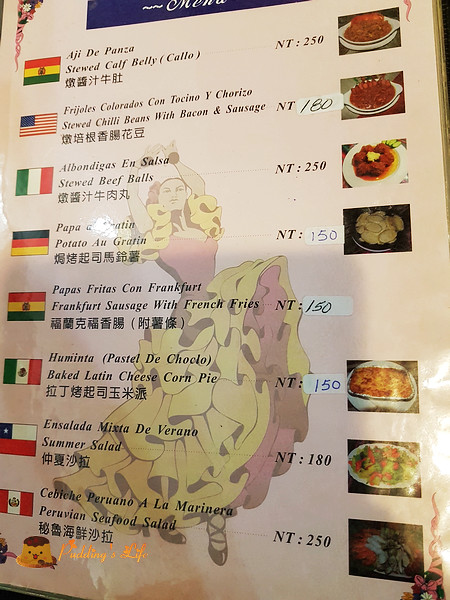This is a detailed menu board at a cosmopolitan restaurant, featuring a diverse range of dishes presented in English and two other languages. The right side of the board prominently displays vivid photographs of various menu items, enticing customers with visual cues. To the left, each dish is described in detail.

At the top of the menu, the first item listed is Stewed Calf Belly, followed by Stewed Chili Beans with Bacon and Sausage. The next dish is Stewed Beef Balls, succeeded by Potatoes au Gratin and Frankfurt Sausage with French Fries. Further down, the menu offers Baked Latin Cheese Corn Pie, a Summer Salad, and a Peruvian Seafood Salad. 

This eclectic assortment of menu options features both familiar dishes and exotic culinary delights from various cultures. Notably, the Frankfurt Sausage with French Fries offers a nod to Peruvian cuisine, while the Baked Latin Cheese Corn Pie draws inspiration from Mexican flavors. This carefully curated menu reflects the restaurant's commitment to bringing a global gastronomic experience to its patrons.